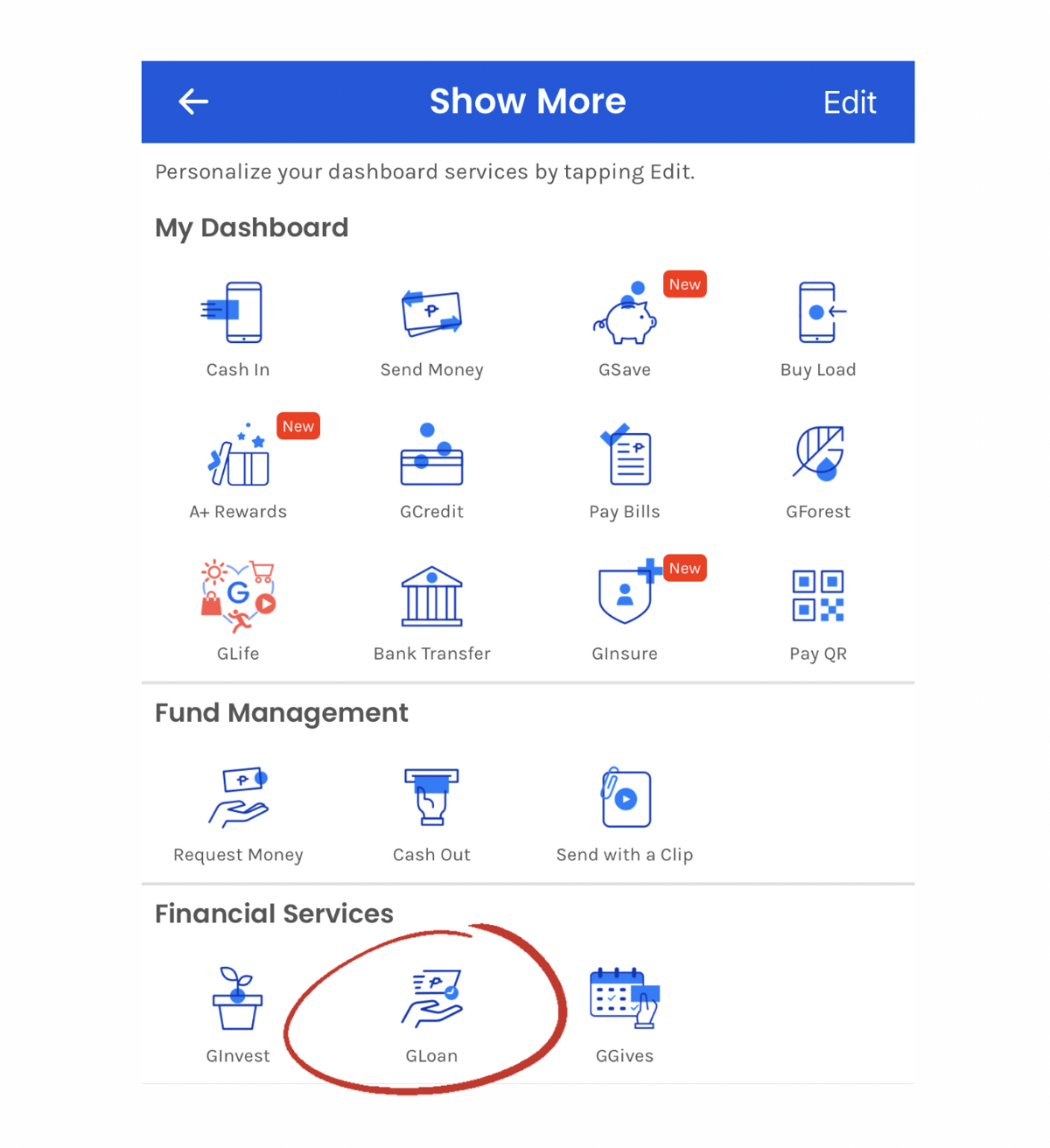In the image, there is a screenshot of a digital dashboard layout. At the top of the interface, there is a box labeled "Show More," followed by an "Edit" button on the right, accompanied by a small arrow icon. Below this, there is a message instructing users to "Personalize your dashboard services by tapping Edit." Directly underneath, the header "My Dashboard" is displayed.

Following this, the layout presents a grid composed of 12 icons arranged in a 4 by 3 configuration. Each icon represents different features and services such as "Cash Ins" and "Money," with descriptive labels below them. The icons are minimalist, outlined in blue, and appear above corresponding text.

Further down, there is a section titled "Fund Management," which mirrors a similar design layout - blue outlined icons above the text labels. 

At the very bottom of the dashboard, there is another section titled "Financial Services." In this section, the service labeled "G Loan" is circled, indicating it as a noteworthy feature or an area of interest in the image.